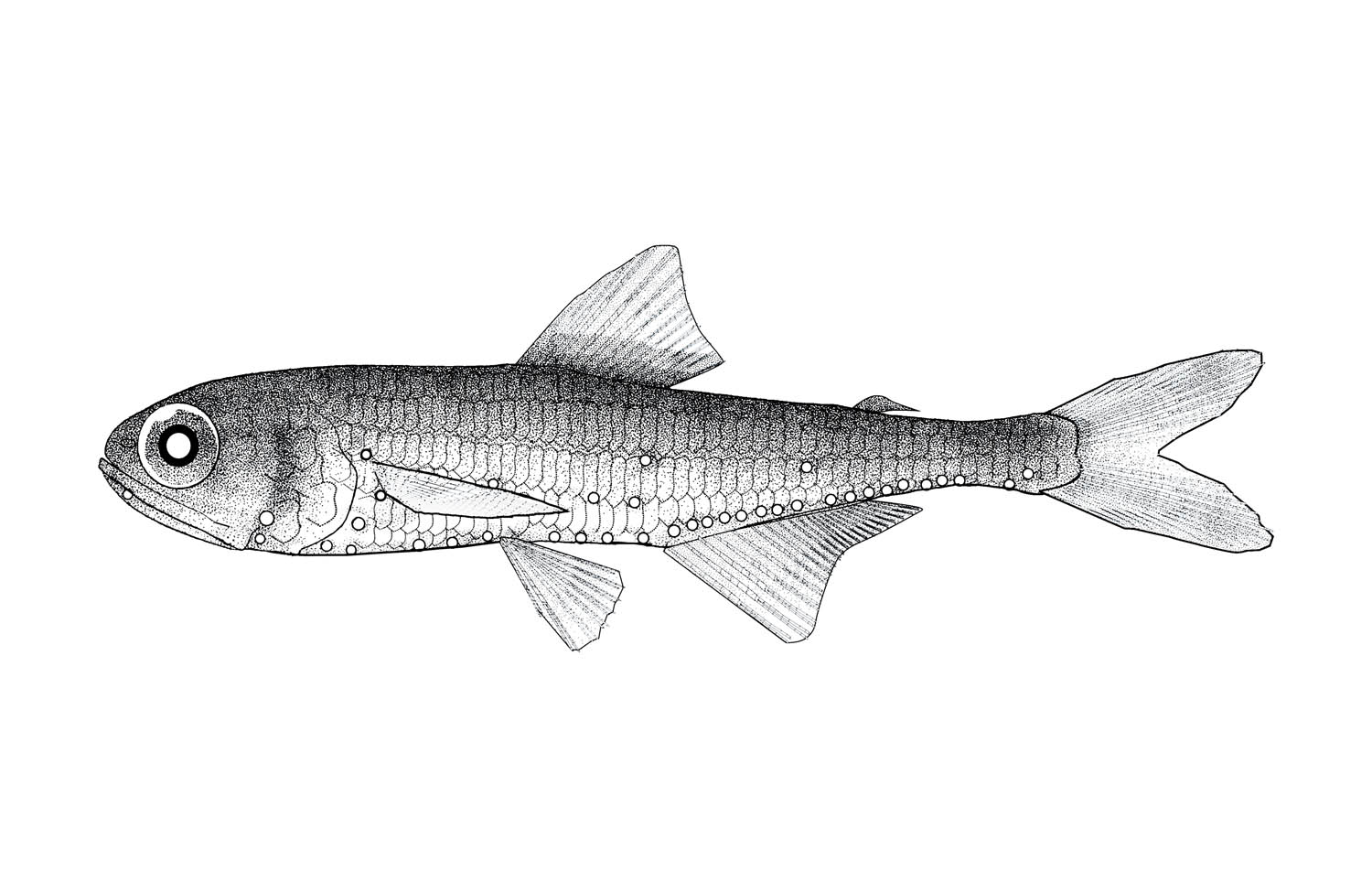This picture is a detailed grayscale drawing of a fish set against a white background. Crafted with charcoal, ink, or regular pencils, the artwork portrays a fish in a side view profile, facing left. The fish’s eye is prominently large and features a white center encircled by a black ring and dotted gray iris, giving the impression it is gazing directly at the viewer. The fish has a typical elongated shape and is rendered in shades of black, white, and gray, with darker tones along its top and belly. Visible scales cover its body, accentuated by many white circles, particularly towards its belly. The fish is equipped with three fins: one dorsal fin, two ventral fins, a pectoral fin, and a tail fin. Additionally, there is a very small dorsal fin located further down its back. This meticulously detailed piece of art captures the intricate details of the fish’s anatomy and texture.